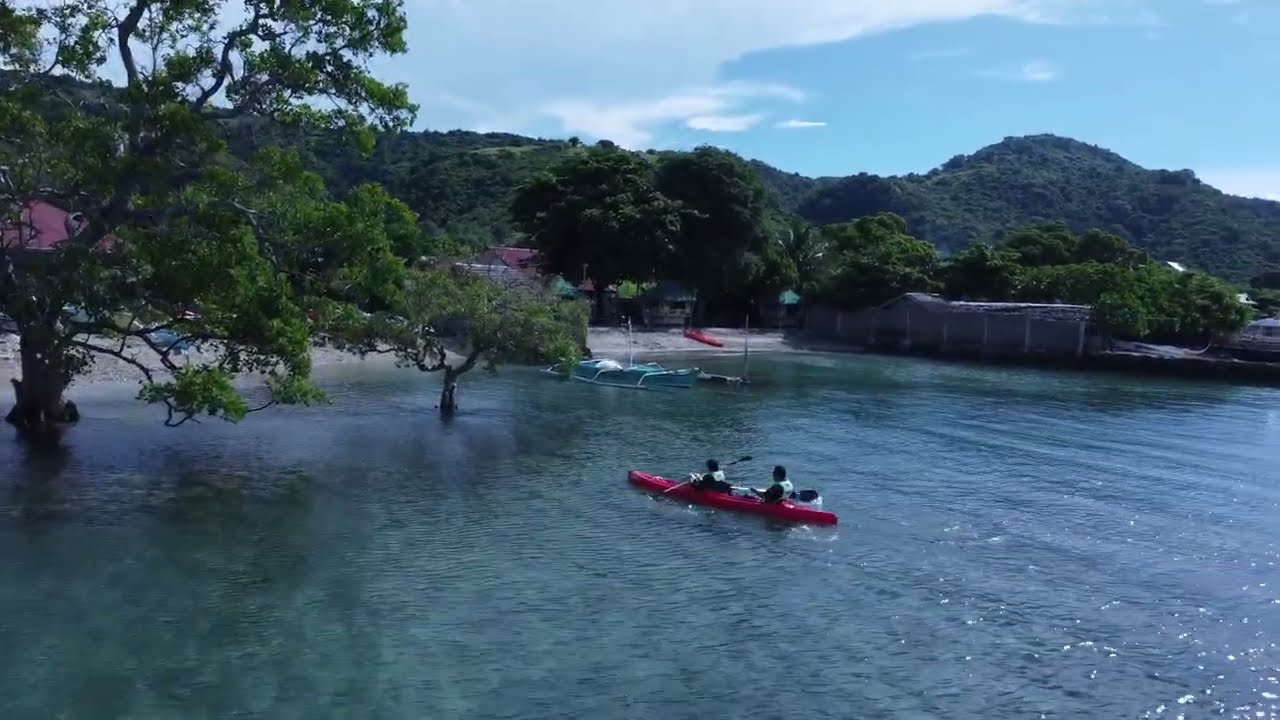In this vibrant outdoor scene, two people are navigating a red canoe on a lake, positioned centrally in the frame. The canoeist at the front is actively rowing with an oar, while the person at the back appears less engaged in rowing, possibly holding their oar lower. The water is near the shore and seems shallow, with deciduous trees emerging directly from it, indicating a higher water level that might suggest flood conditions. Surrounding the water, which occupies the bottom half of the image, are patches of shoreline with some houses and possibly a business where boats are docked. In the background, lush green mountains and hills rise up under a clear, blue summer sky dotted with a few clouds. To the right, foliage from a nearby tree dips into the frame, adding a natural, leafy border.